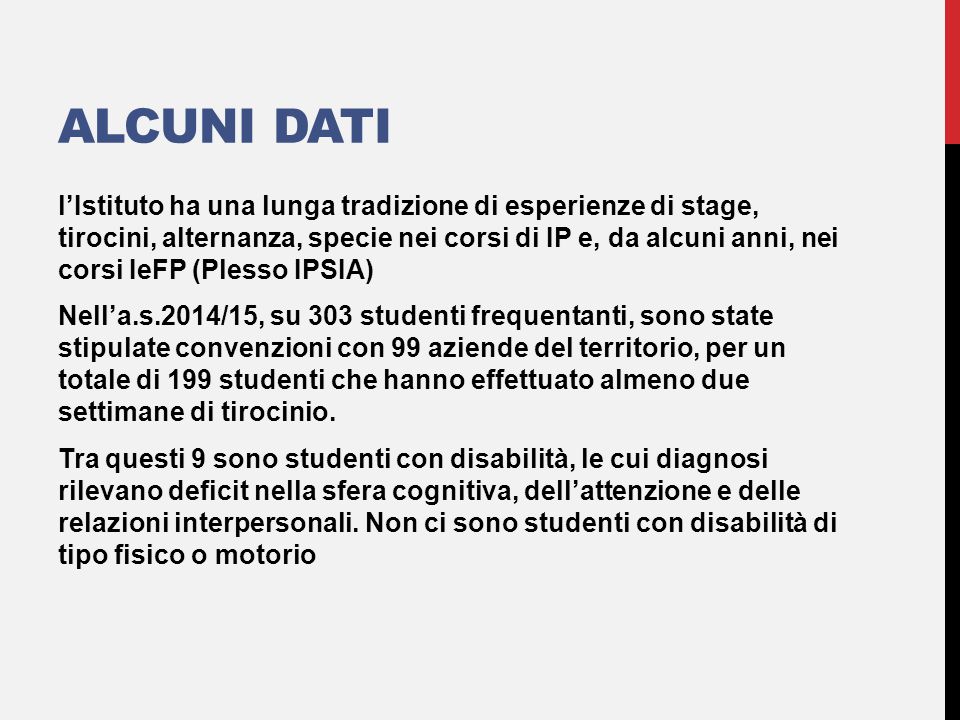The image is a presentation slide with a white or gray background, featuring a blue header text that reads "Alcuni Dati" (Italian for "Some Data") in large font at the top left. The rest of the text, which is in black and aligned to the left, is detailed in Italian. The slide contains information about internships and educational programs. Specifically, it refers to the 2014-15 school year, indicating that out of 303 students, agreements were made with 99 local companies for a total of 199 students to complete at least two weeks of internship. Among these, 9 students have cognitive, attention, and interpersonal relationship deficits, with no students reporting physical or motor disabilities. On the far right of the slide, there is a decorative vertical bar with a gradient, starting red at the top and transitioning to black towards the bottom.